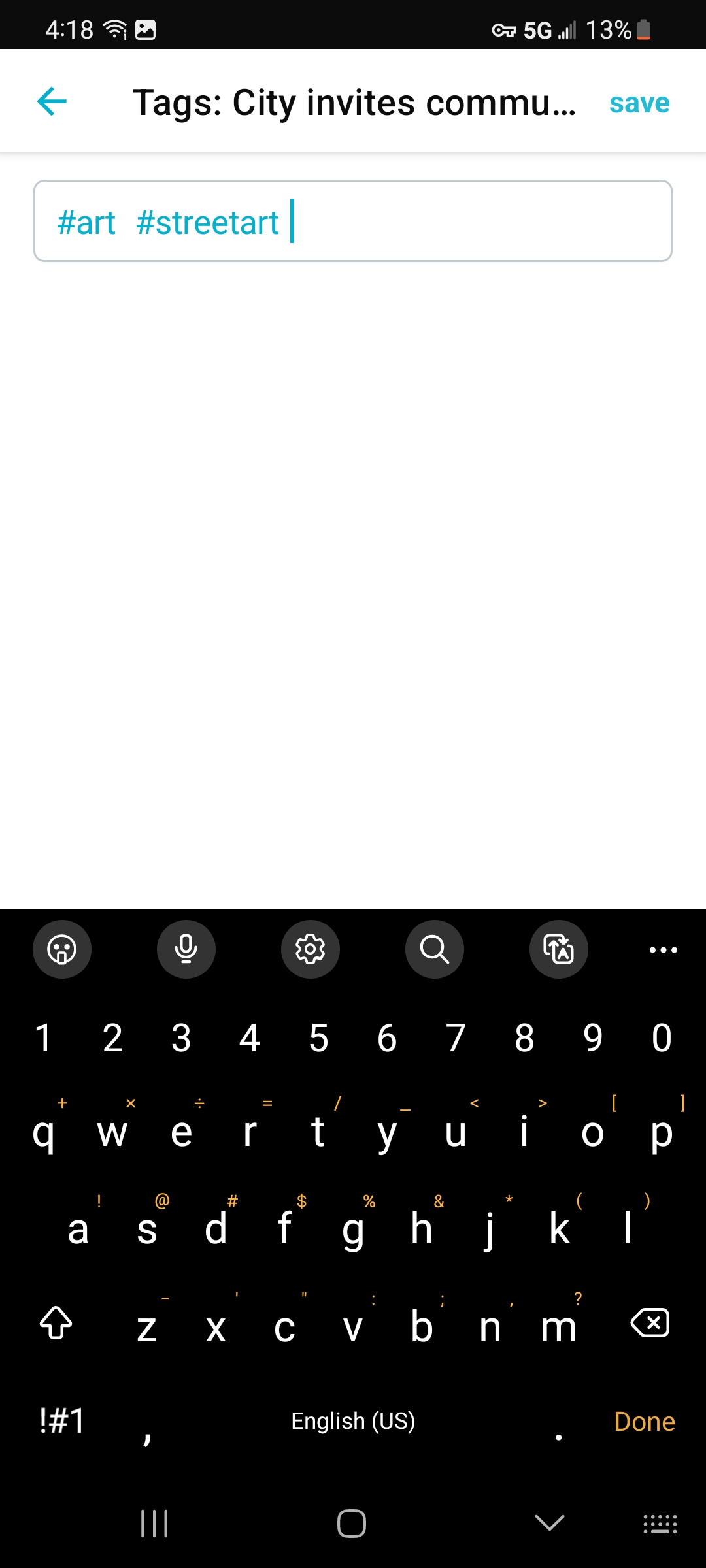The screenshot showcases various elements of a mobile interface with striking details:

At the very top, there is a black status bar displaying the time as 4:18. It also includes icons for Wi-Fi, 5G signal strength, and battery life indicating 13% with a red low battery icon. Below the status bar, the screen transitions into a white background.

Toward the upper center, there is a tealish-light blue arrow against the white background, pointing downward. Directly beneath, black text reads "city invites Kamu CLM you," though the text is partially cut off. A blue "Save" button is positioned alongside this section.

Further down, there is a search box with a grey outline. Inside the box are hashtags #art and #streetart, displayed in a Tiffany blue color.

Beneath the search box, there is a blank white square space, possibly for image or text input. 

Continuing down, a black keyboard occupies the lower part of the screen. The keyboard features white letters and numbers, while special characters are indicated in an orange color. The "Done" button near the top of the keyboard also appears in orange. Above the keyboard, there are several icons: an emoji face, a microphone, a cogwheel, a magnifying glass, and some sheets of paper with the letter 'A' on them. Additionally, three white dots are present.

At the bottom of the keyboard, four smaller icons are visible: three horizontal lines, a square, a down arrow, and a mini keyboard icon.

Overall, no specific actions or gestures are captured in this otherwise static screenshot, which provides a comprehensive view of the mobile interface details.